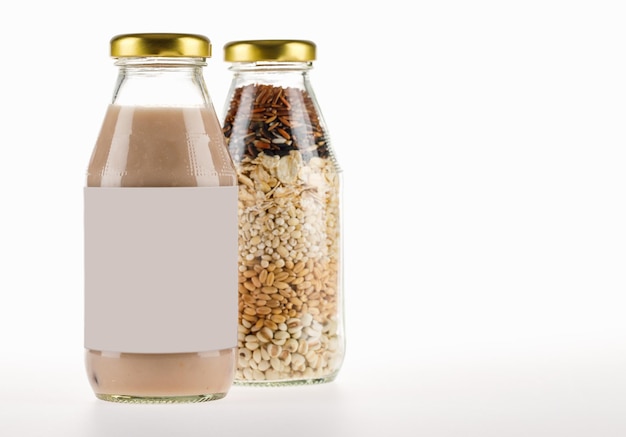The image displays two clear, short, and slightly bulbous glass bottles with gold caps, positioned against a white background with a light-reflective surface. The bottle on the left is partially in front of the bottle on the right, with a wide gray label that nearly spans from the neck to the base. This bottle contains a brown liquid resembling chocolate milk. The bottle on the right, although partially obscured, is filled with an assortment of layered nuts and seeds. The layers from bottom to top consist of white nuts, possibly pistachios, followed by lighter tan seeds, darker small grains, and then a mix of dark brown and lighter grains at the very top. This arrangement highlights detailed textures and colors within the clear glass.